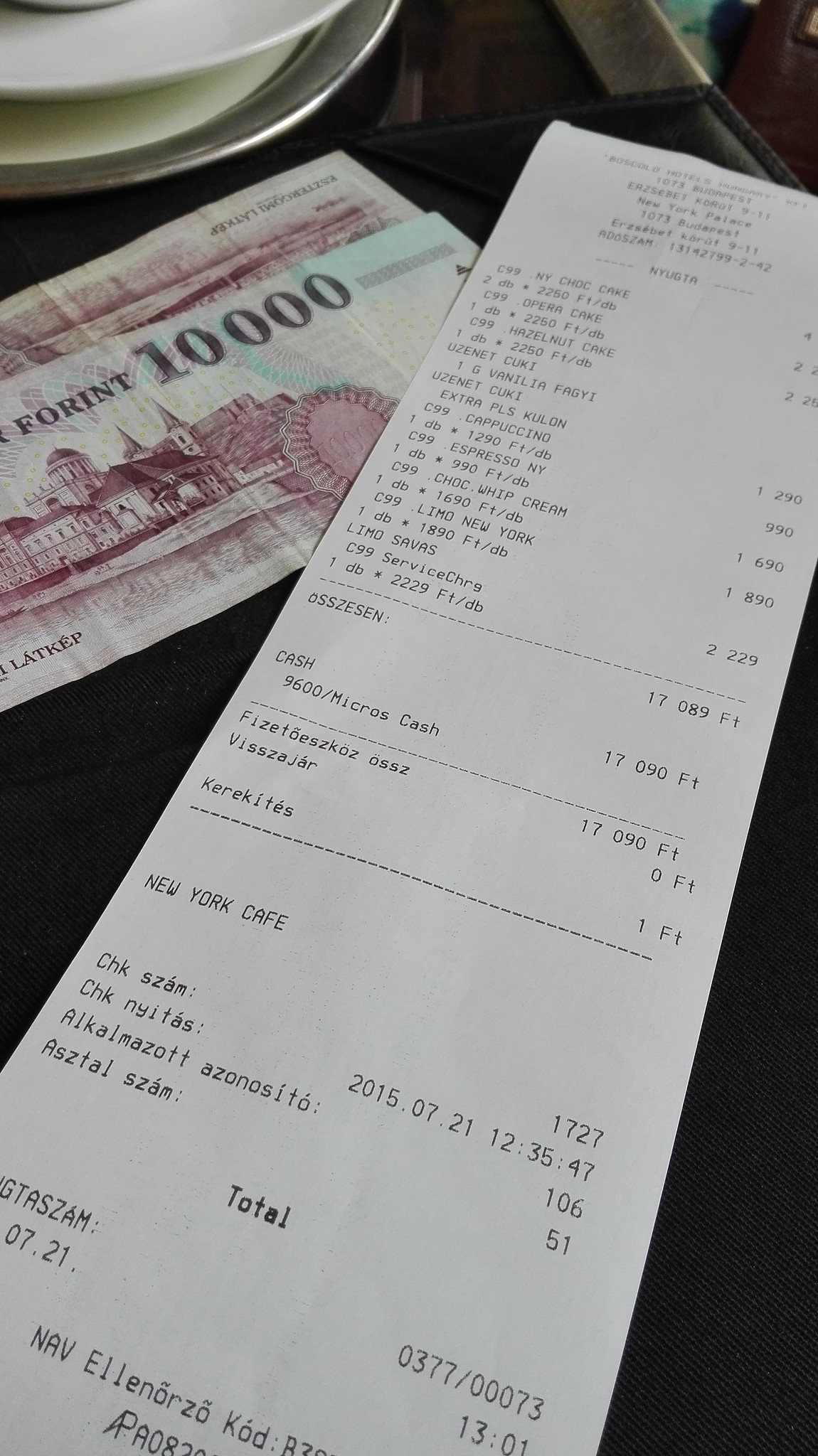The image showcases an overhead view of a black leather table adorned with a receipt from New York Cafe, located at New York Palace, 1073 Budapest. The white receipt, written in Hungarian with some English items, lists New York chocolate cake, opera cake, and hazelnut cake, with a total amount at the bottom. Positioned to the right of the receipt are two pieces of Hungarian currency, notably a 10,000 forint bill with a white and pinkish interior and an image of a city in pink. In the top left corner of the image, there’s a plate with a metal rim and a white porcelain interior. The receipt and currency stand out vividly against the black leather backdrop.